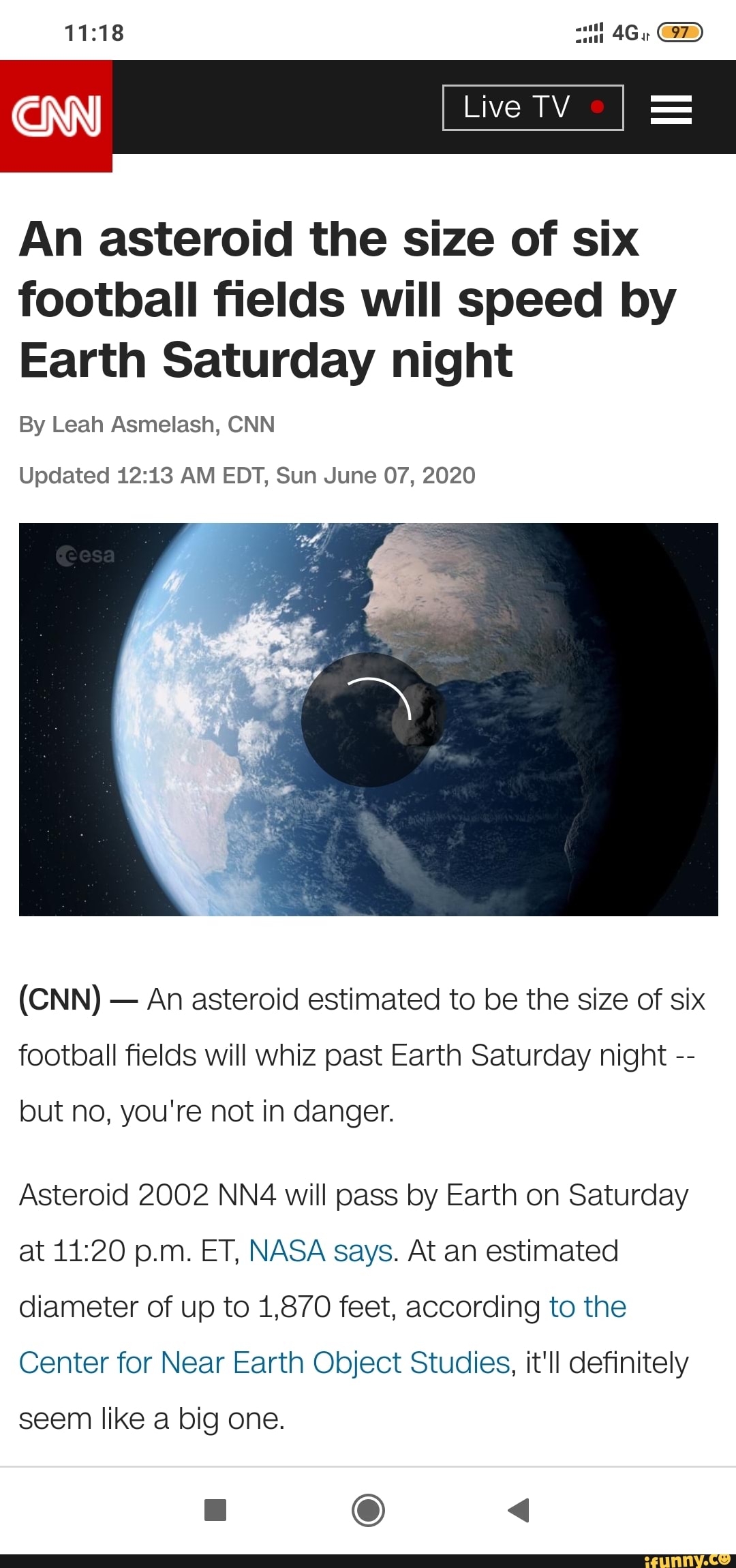In the image, the time is displayed as 11:18, with a 4G signal indicator and a yellow horizontal battery icon showing 97% on the right side. Below this, a red box with "CNN" is prominent, alongside a long black box containing "Live TV." Beneath these elements, the main news headline reads, "An asteroid the size of six football fields will speed by Earth Saturday night," authored by Leah Asmelash. It notes an update at 12:13 AM EDT on Sunday, June 7th, 2020. 

The visual centerpiece of the image is a picture of Earth, predominantly blue and white, set against a black background. Below this, in parentheses, is the text "CNN." The first paragraph of the news article states, "An asteroid estimated to be the size of six football fields will whiz past Earth Saturday night, but don't worry, you're not in danger." The following text details that "Asteroid 2002 NN4 will pass by Earth on Saturday at 11:20 PM," according to NASA, with an estimated diameter of up to 1,870 feet as reported by the Center for Near Earth Object Studies, shown in blue text. The text ends with a note highlighting the sizable nature of the asteroid.